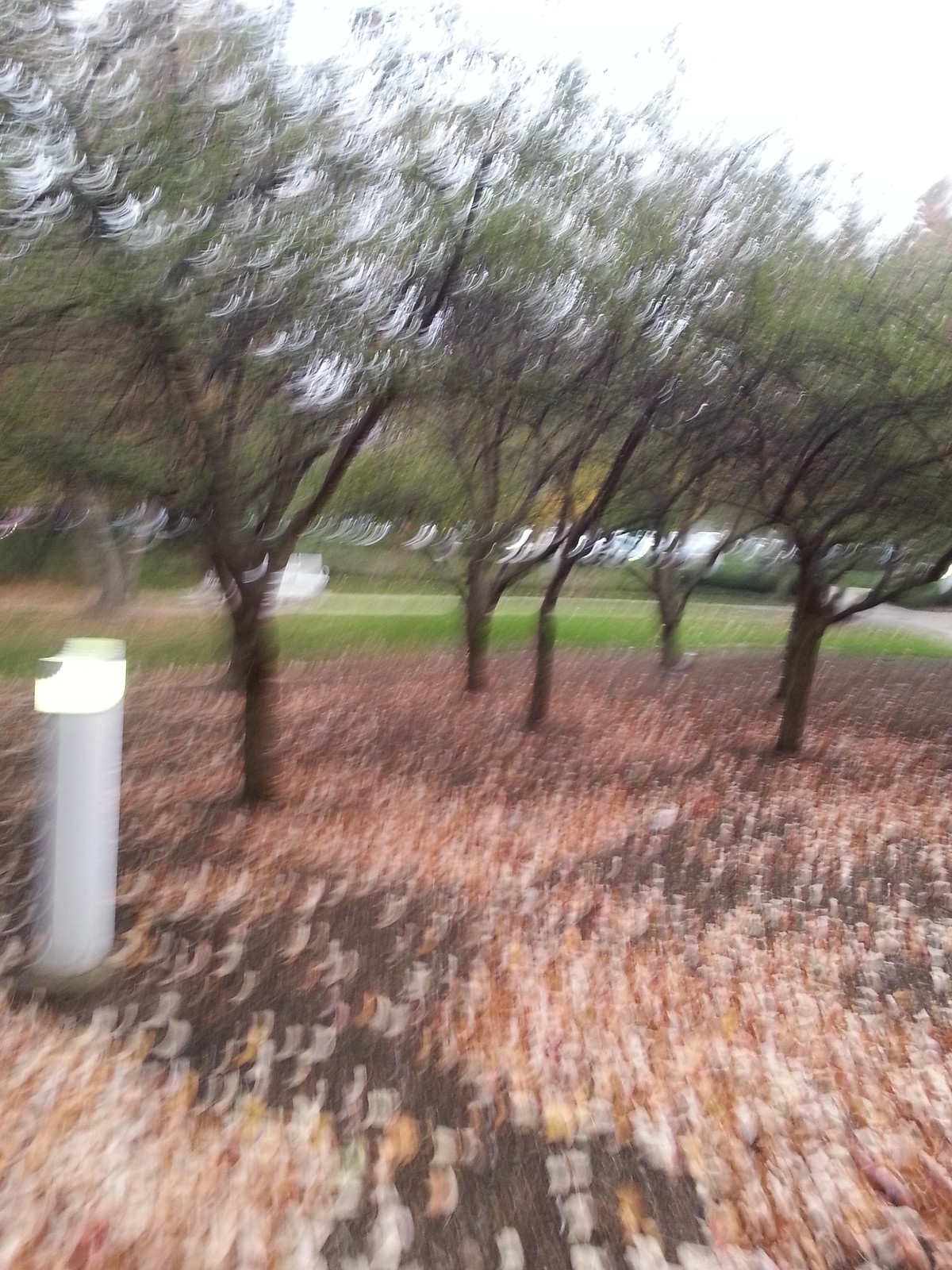This photograph captures a tranquil park scene featuring a mulched clearing dotted with approximately six or seven trees, each spaced evenly apart. Fallen, dried leaves cover the ground, adding a seasonal touch to the image. In the foreground to the left, there is a white utility box, which stands out against the natural surroundings. The picture is somewhat blurry, giving it a nostalgic, almost dream-like quality.